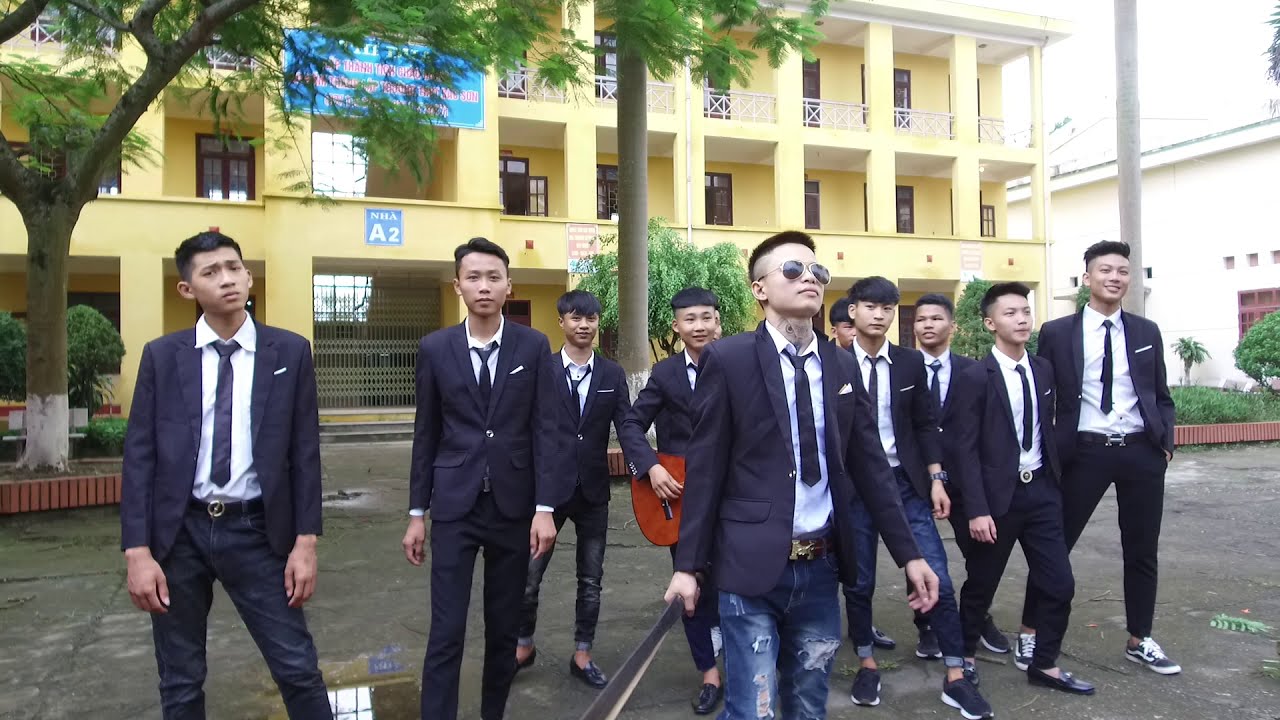A group of twelve young Asian men are standing together on an asphalt surface in front of a tall three-story yellow building. They are all dressed in blue blazers with white button-up shirts, dark ties, and most are wearing blue jeans. The young man standing furthest in the front, who looks to be the lead, is distinctively wearing blue jeans with white holes and sunglasses, giving him a cool, standout appearance. He is holding something that resembles a sword or a stick, adding an interesting dynamic to the scene. Another young man behind him is holding a guitar, suggesting the group might be a band. They display a mix of expressions; some are smiling while others look serious, and their gazes are mostly directed slightly to the right. 

The yellow building behind them has two sets of balconies, the lower one with a yellow base and the upper one bordered by white railings. The presence of windows within the balconies is noticeable. To the left side of the image, there's a tree with white paint at the base of the trunk and green leaves that spread out over part of the group. In the distance on the far right, a white building is visible through a light haze, and there are puddles on the ground indicating a recent rainfall. The scene seems to be outdoors, possibly in a parking lot, with the setting suggesting a mix of suburban and urban elements.